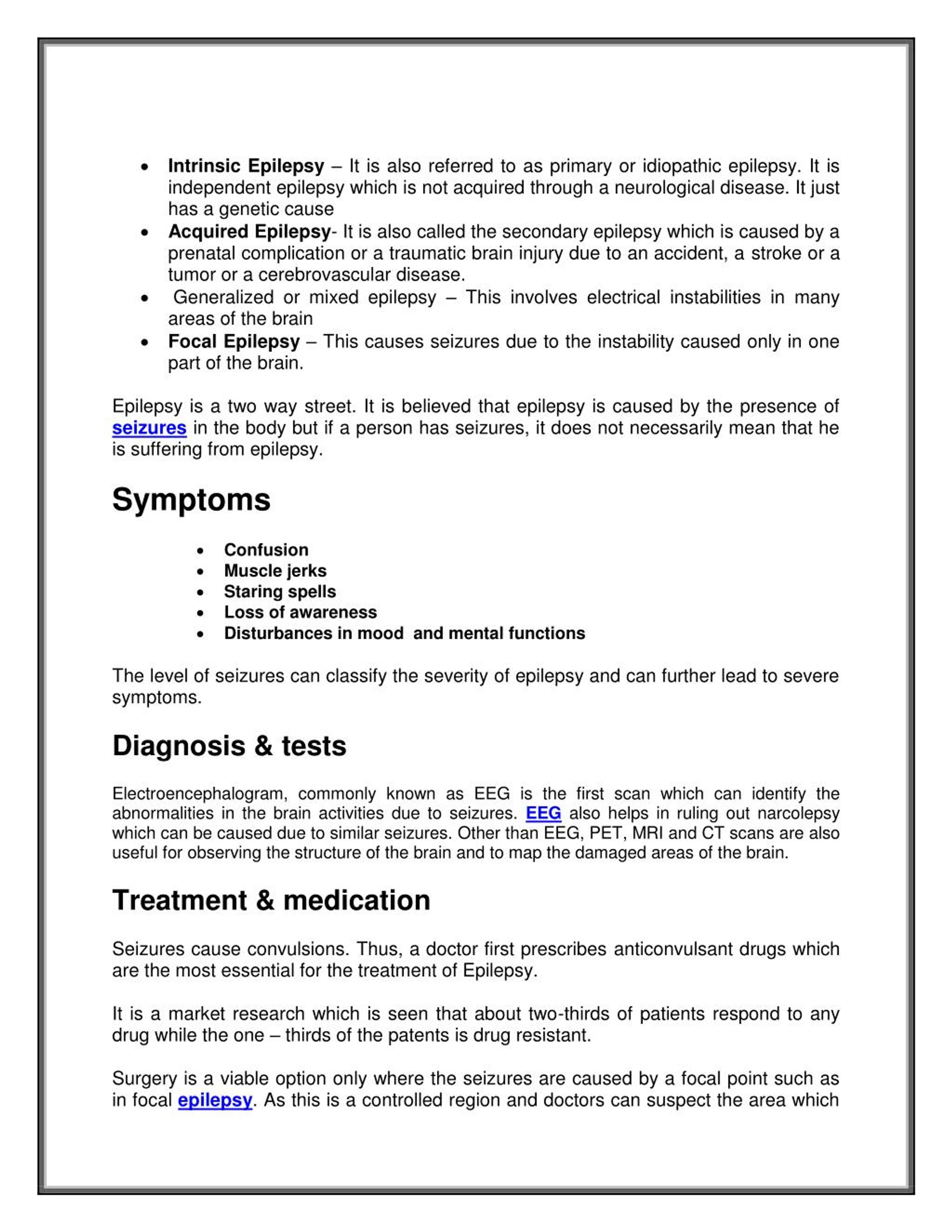This image depicts a typed page discussing different forms of epilepsy, suggesting it is part of a larger document. The content begins with a bullet point:

- **Intrinsic Epilepsy**: Also referred to as primary or idiopathic epilepsy. This type of epilepsy is not acquired through any neurological disease but has a genetic cause.

- **Acquired Epilepsy**: Also known as secondary epilepsy, it results from prenatal complications or traumatic brain injuries caused by accidents, strokes, tumors, or cerebrovascular diseases.

The page further elaborates on other forms of epilepsy:

- **Generalized or Mixed Epilepsy**: Characterized by electrical instabilities in multiple areas of the brain.
- **Focal Epilepsy**: Causes seizures due to electrical instability confined to one part of the brain.

Additionally, the text addresses the nature of epilepsy, describing it as a "two-way street." It explains that while epilepsy is caused by the presence of seizures, not every person who has seizures necessarily suffers from epilepsy.

Following this explanation, the page lists symptoms, provides sections for diagnosis and tests, and outlines treatment and medication options.